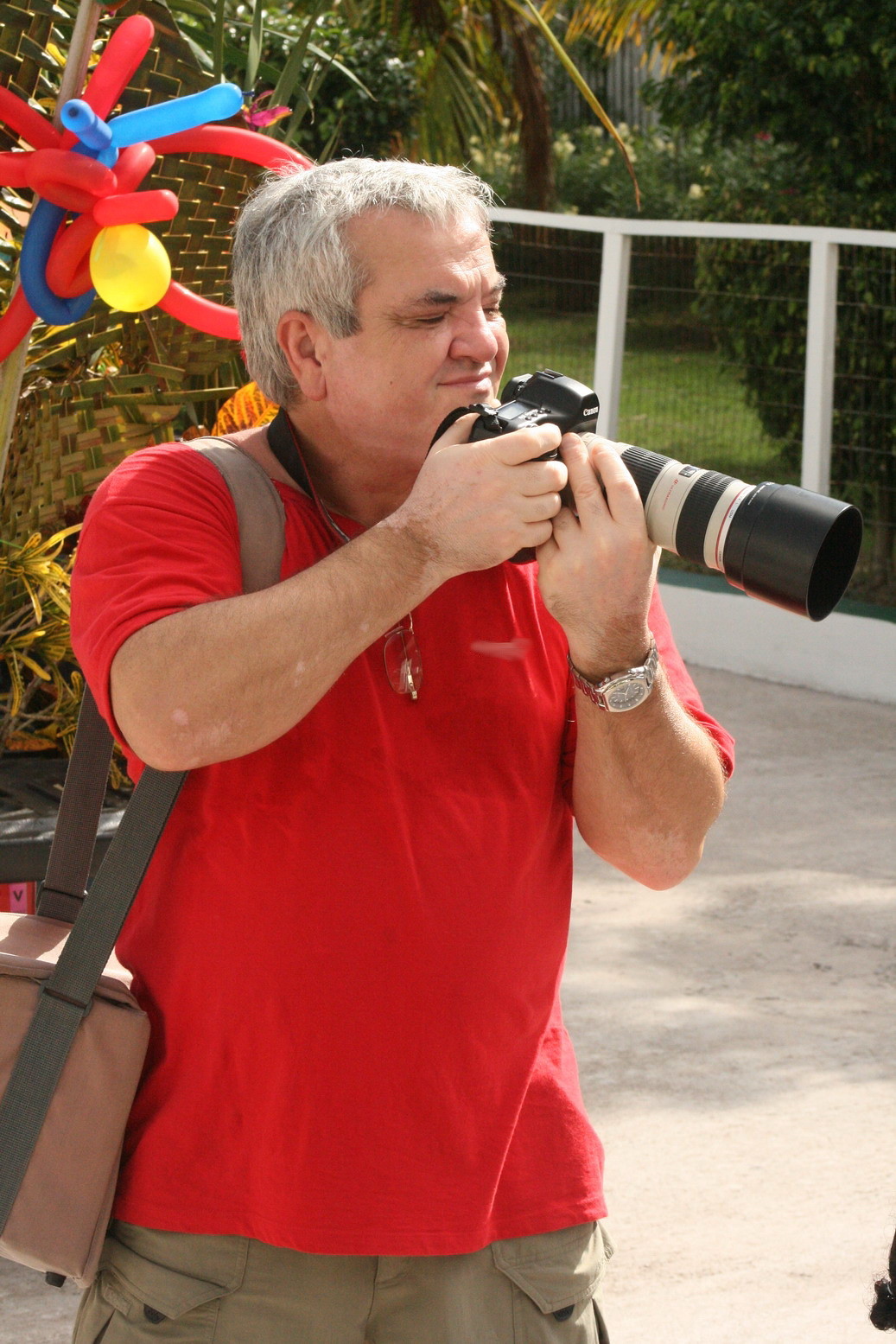The photograph captures an older Caucasian man, shown from the waist up, immersed in his photography. He is dressed in khaki pants and a medium red short-sleeve shirt, with a gold watch visible on his left wrist. A brown-strapped bag, likely a camera bag, hangs from his right shoulder. His mostly gray hair, with hints of black, frames a face focused intently on the task at hand.

The man is two-handedly holding an SLR camera equipped with a telephoto lens and a lens shade, aimed slightly out of the frame to the left. His lips are pursed as he peeks through the viewfinder, positioning the camera about chin height, with his right hand gripping the side and his left hand steadying the lens.

The background hints at an outdoor setting, featuring palm tree leaves and a white fence interspersed with metal crossbars. Festive balloons float behind him, suggesting he might be at a public event or celebration, perhaps a zoo or a birthday party. The scene exudes a casual yet focused atmosphere, capturing the man in the midst of his photographic pursuit.